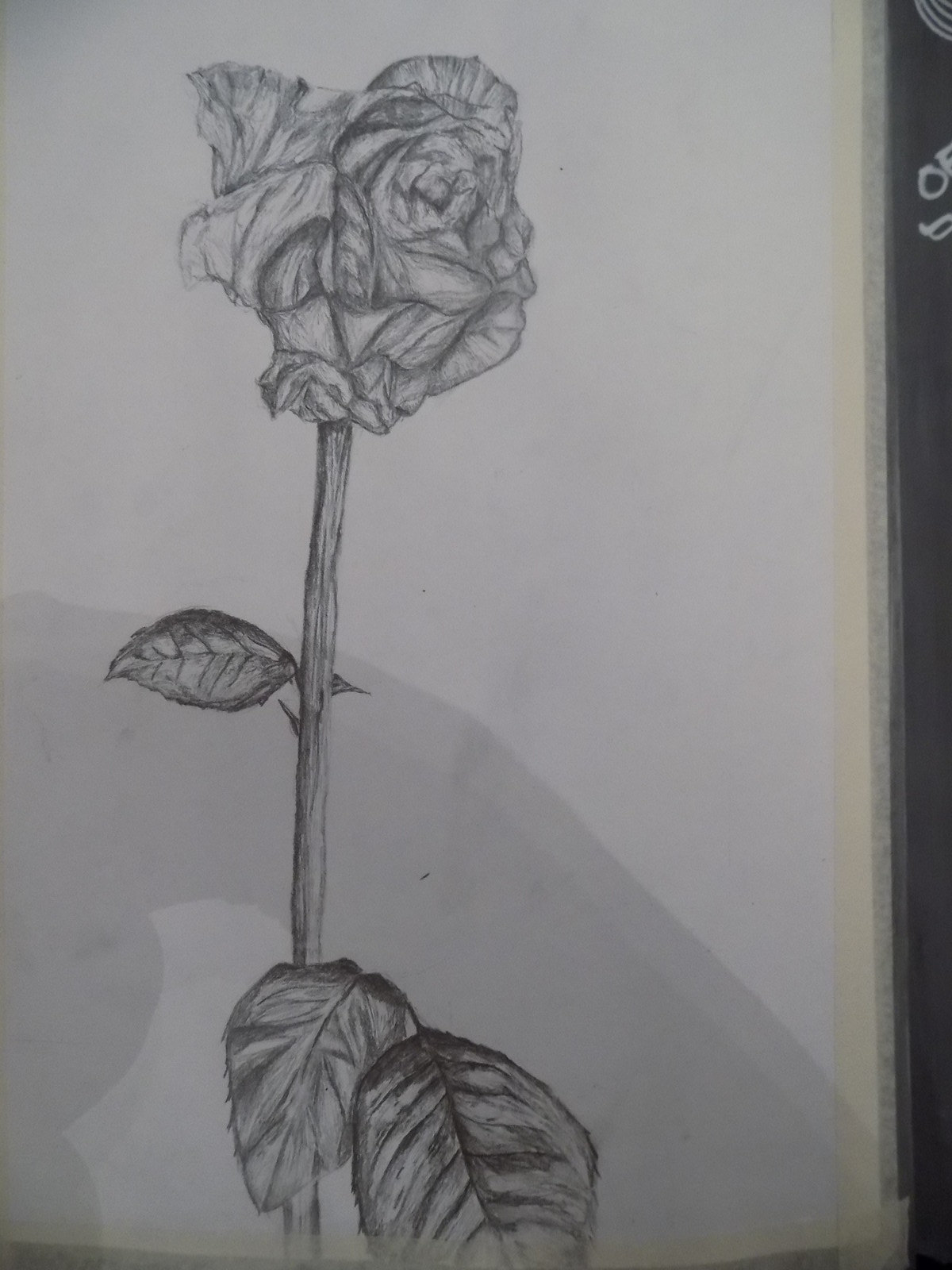This detailed pencil sketch, centered on a single, fully-bloomed rose, is meticulously hand-drawn on a piece of white paper, possibly torn from a sketchbook. The paper appears to be loosely taped down onto a black surface, casting a faint shadow below that may resemble an arm. The rose's abundant petals are intricately articulated, encircling the central bud and exhibiting slight crinkling at the edges, hinting at a mature bloom. The tall, vertical stem of the rose is studded with two sharp thorns halfway up and features a small leaf hanging from the left side. At the base of the stem, two larger, lush leaves emerge, pointing downward, with their veins carefully rendered in pencil. The sketch is densely shaded throughout, emphasizing the three-dimensionality of the rose and making the delicate yet prickly nature of this botanical subject vividly clear.